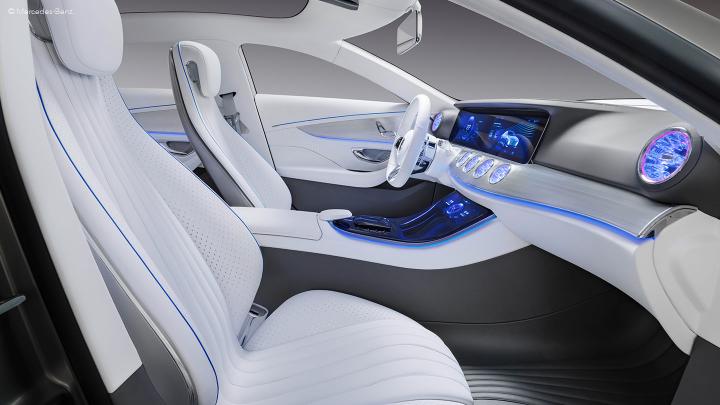This image depicts a modern, possibly futuristic, automobile interior characterized by a predominantly white color scheme, which extends to the seats, steering wheel, and various dashboard components. The dashboard features darker elements, including large, circular readouts reminiscent of aviation instruments, and an array of data displays in blue and black hues. The steering wheel, which appears smaller in circumference, is positioned against a steeply angled, aerodynamic front section. The photo is taken from the passenger side with the door open, offering a clear view of the two front seats and part of the rear cabin, all clad in white with gray backs. Notably, the dashboard and driver's door emit soft blue and purple lights, enhancing the vehicle's sleek, high-tech atmosphere. The car seems compact, indicated by the tight headroom and the appearance of small doors. This detailed interior view, with its clean lines and state-of-the-art features, suggests a newly designed, high-end sports car or luxury vehicle.